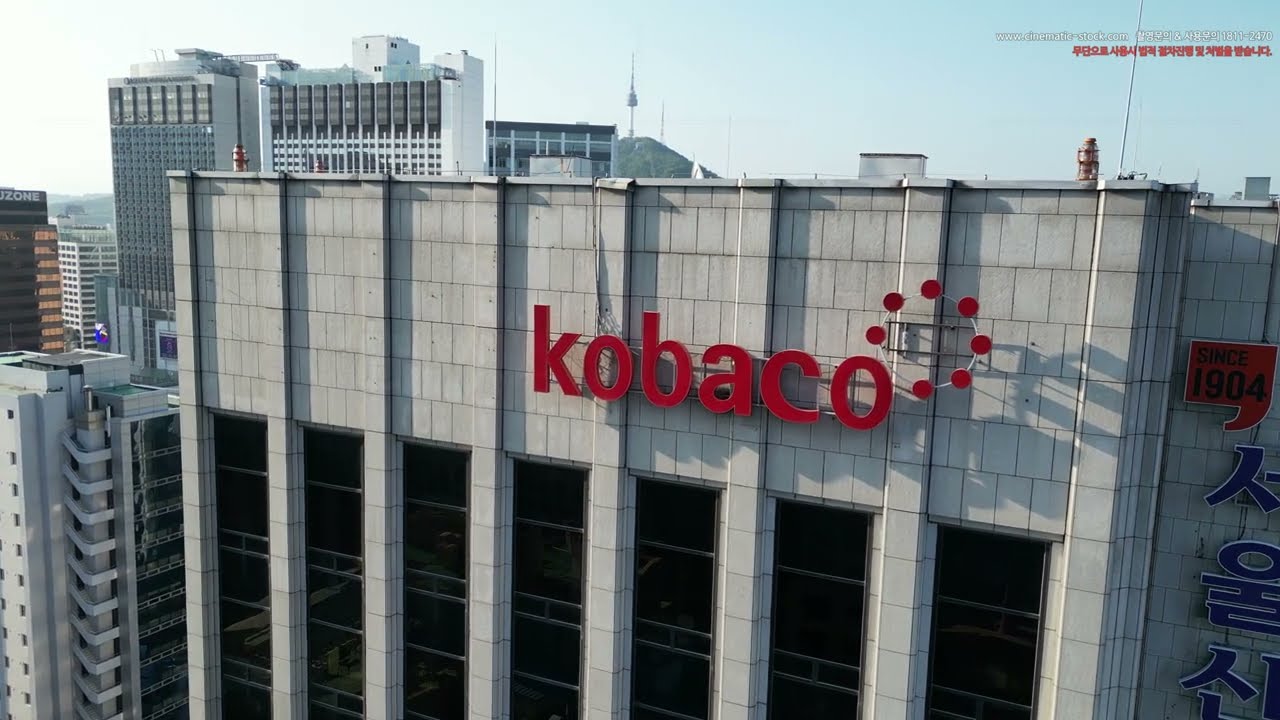This outdoor photograph, taken on a clear day, features a tall building in a major city, constructed primarily from white concrete blocks and gray square stonework. The structure prominently displays the name "Kobaco" in bold red font, accompanied by a circle made of smaller red dots. The building is multi-storied, with its top floors constructed from cement blocks and the lower sections from glass panels separated by cement pillars. There are seven vertical lines of dark, possibly black, windows along the building. To the right side of the building, Chinese characters run vertically in blue. The top right corner of the image contains some Chinese text on two lines, with the top line in white font and the bottom line in red font. In the background, additional, taller skyscrapers are visible, adding depth to the cityscape, while a clear blue sky stretches above.